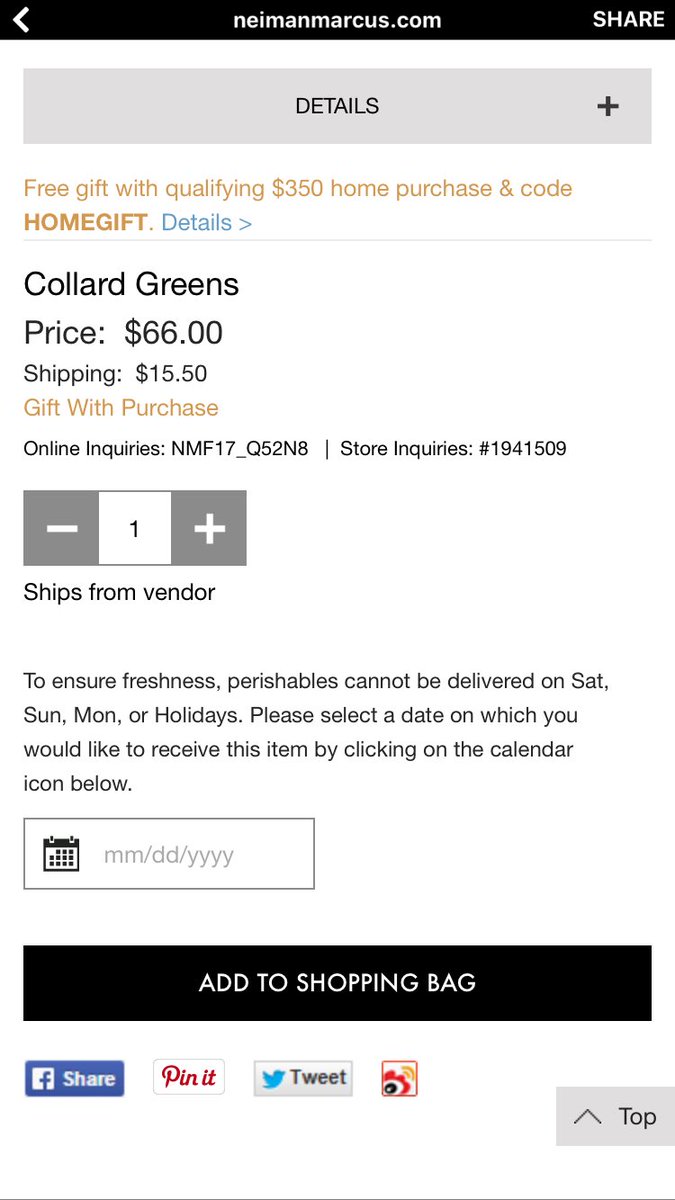This is a screenshot from the Neiman Marcus website displaying a product page. At the top of the page, the black header features the Neiman Marcus logo and "neimanmarcus.com." To the left, there is a left-pointing arrow, and on the right, there is an option labeled "Share."

Further down, there is a gray box titled "Details" with a plus sign to its right. The page advertises a "Free Gift with a Qualifying $350 Home Purchase" using the code "HOMEGIFT." The word "Details" is highlighted in blue with a right-pointing arrow beside it.

The featured product is "Collared Greens" priced at $66 with an additional shipping cost of $15.50. There is an orange highlight stating "Gift with Purchase." For online inquiries, a specific code is provided, and for store inquiries, another code is given. The note "Ships from Vendor" is also mentioned.

Below, there is a quantity selector with a default value of one, a negative sign to decrease and a positive sign to increase the quantity. There's an advisory that perishables cannot be delivered on Saturday, Sunday, Monday, or holidays to ensure freshness. It instructs the user to select a delivery date by clicking on a calendar icon that allows selection by month, date, and year.

Near the bottom, there is a black rectangular button with "Add to Shopping Bag" written on it. Below this, sharing options are listed including "Share" in blue, "Pin it" in red and white, "Tweet" in blue, black, and white, and an icon with red and yellow colors.